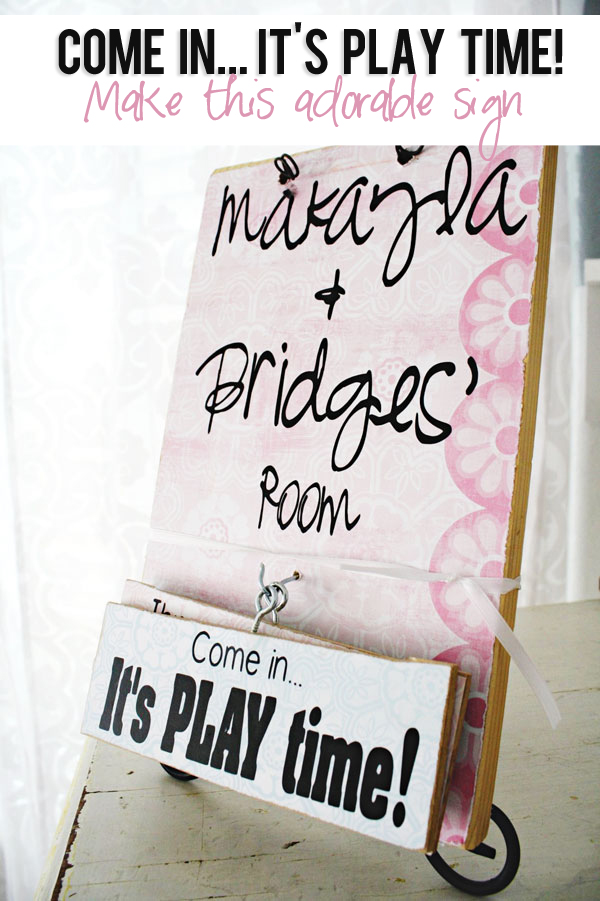The image is a close-up, rectangular photograph of a wooden sign taken indoors during daytime, with sunlight streaming through a light-colored curtain with a faint blue print, suggesting a cheerful ambiance. At the very top of the sign, a white banner runs left to right featuring bold, black text that reads "Come in... It's playtime!" Below this, in pink text, it says, "Make this adorable sign." The main sign beneath this has a light pink background with black lettering that reads "Makayla + Bridges' Room." The sign is mounted on a white, slightly chipped wooden surface, adding a rustic touch. Attached to the bottom of the main sign, there's a metal hook with two smaller signs hanging from it. The top smaller sign also reads "Come in, It's playtime!" while the text on the sign behind it is obscured. Adjacent to the sign on the left side of the image is a light-colored curtain, and the entire setup seems to be placed on wooden flooring that’s painted white and showing wear.